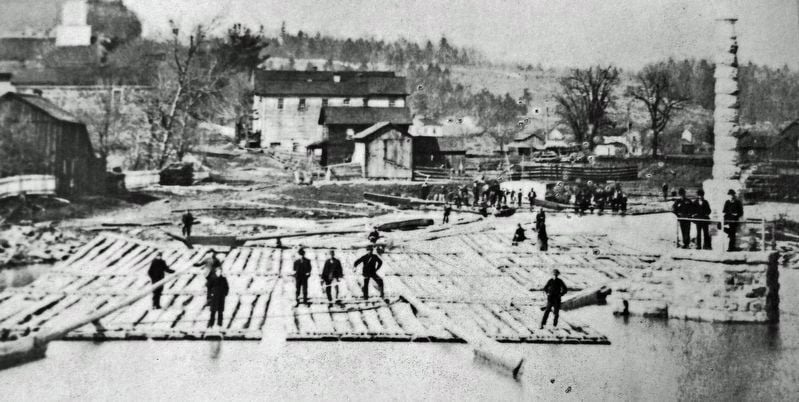This vintage black and white photograph depicts a bustling, historical riverside scene, likely from the late 1800s or early 1900s. Numerous men, all dressed in black clothing and most donning hats, are standing on flat wooden barges fashioned from logs, floating on a shallow river. A long oar in the center of each barge hints at their use for steering. One gentleman on the leftmost barge is actively holding the oar, while others stand still, seemingly posing for the photograph. To the right, a stone deck or tower stands elevated, with a few individuals posing around it, observing the scene below. Background details reveal a landscape of bare-branched trees, indicative of winter, and a hillside dotted with pine trees. Several rustic buildings, including an old stone mill and barns, complete the picturesque backdrop. The grainy image quality and lack of color further emphasize the antiquity of the scene.